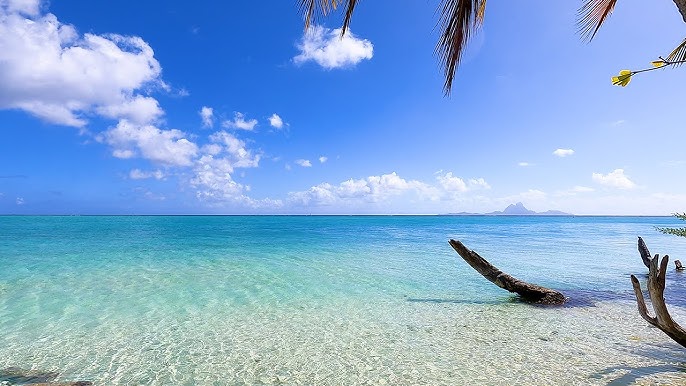The image depicts a serene beach scene featuring a crystal-clear, blue ocean transitioning from light, sandy hues near the shoreline to a deep, rich blue in the distance. The sky above is mostly a clear blue adorned with occasional fluffy white clouds, contributing to a tranquil atmosphere. In the distance, a silhouette of a mountain range, possibly including an extinct volcano, adds a dramatic backdrop, with the mountains casting a bluish hue. The sandy beach in the foreground is pristine and white, scattered with elements of driftwood and branches, punctuated by patches of yellow flowers and green foliage. At the top edge of the image, partially cut-off leaves of a palm tree dangle into the scene, enhancing the tropical feel. To the far right, the shore gently curves, where one can just make out the gentle waves lapping against the sand. The overall composition is one of natural beauty and calm, inviting the viewer to wade into the clear waters and enjoy the idyllic setting.